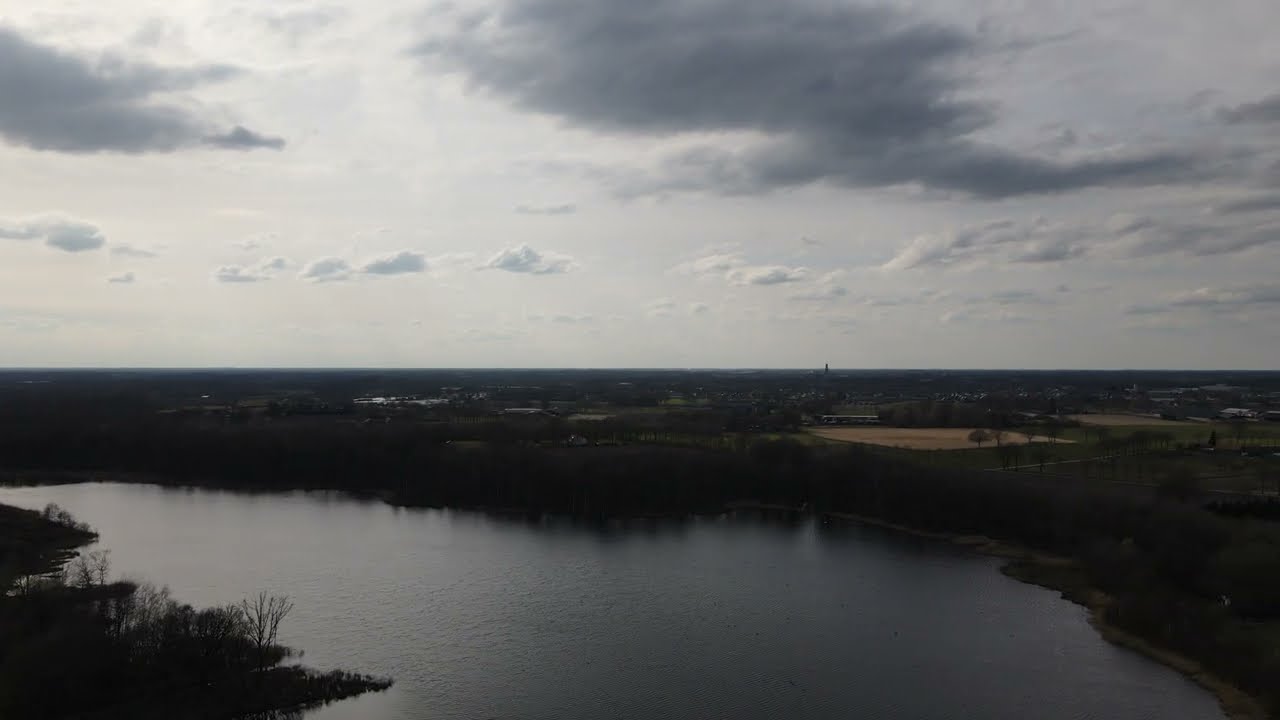This aerial photo, likely taken by a drone, captures an expansive landscape during what appears to be an overcast late afternoon or near sunset. The central focus is a dark, opaque lake that stretches across the bottom center of the frame, flanked by fluffy, fern-like trees lining its entire edge. Surrounding the lake is a vast, sandy area leading to dense greenery, with a straight trail or sidewalk running parallel to the shoreline and extending into the distance. The overcast sky is dominated by thick, dark gray clouds, with one lighter area in the top left where some sunlight seeps through. The horizon is flat and marked by a few distant buildings with white roofs, barely visible, alongside a tall tower that rises prominently above the landscape. Additionally, a train appears to be moving across what seems to be a train track near the sandy area, adding to the serene and expansive atmosphere of the scene.